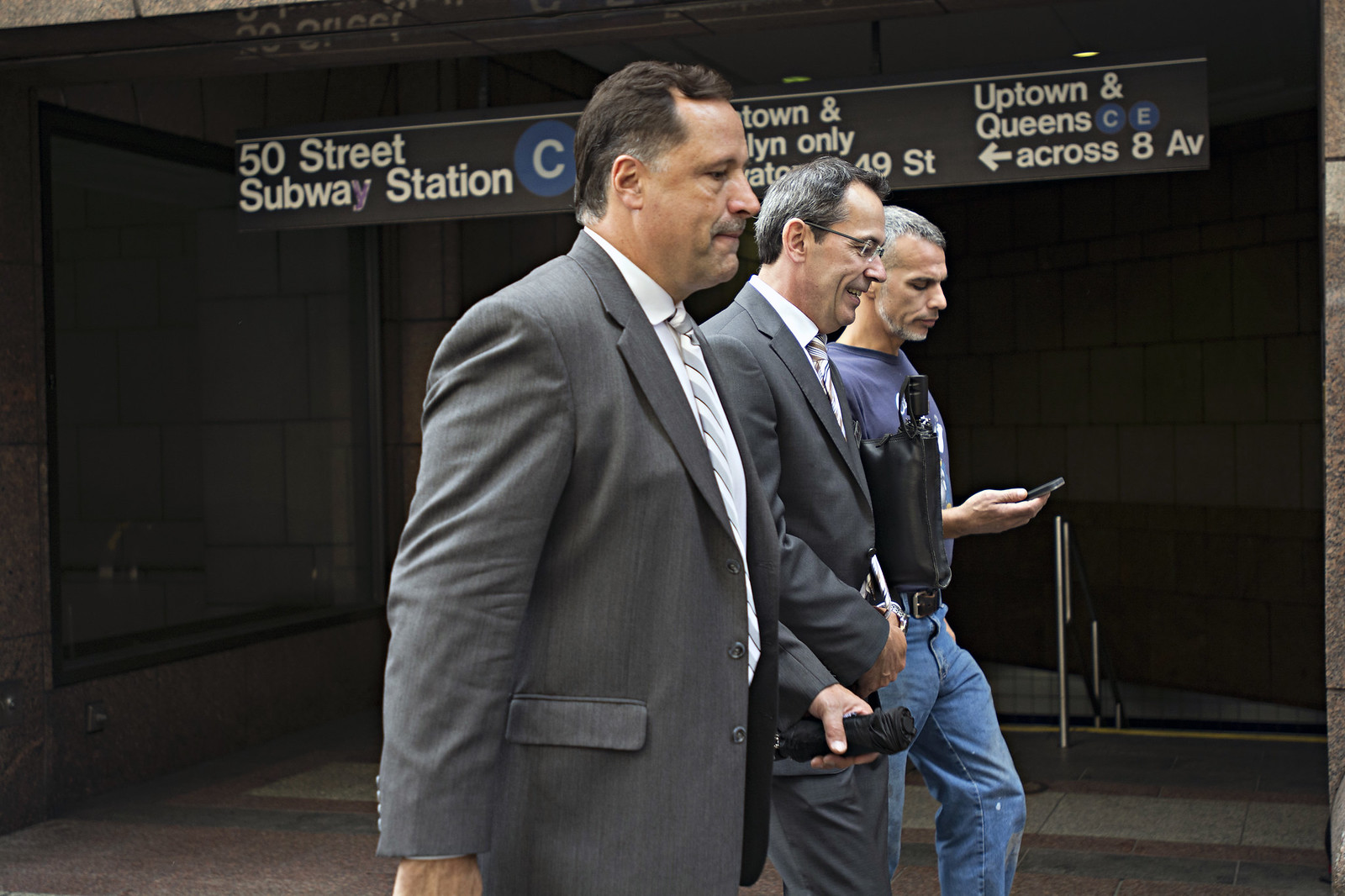In this detailed photo taken in New York City, just outside the 50th Street subway station entrance for the Uptown and Queens C and E lines across 8th Avenue, three men are walking from left to right along a sidewalk. The man closest to the camera is dressed in a gray suit, complemented by a white shirt and a striped gray and white tie. He is partially visible from the waist up and appears to be carrying a folded umbrella in his left hand. The middle man, also clad in a suit and tie, is distinctively smiling and appears to be holding his hands together in front of him, which adds an air of mystery as if he were in handcuffs though none are visible. Both men in suits lend a formal flair to the image. The third man, positioned furthest away, contrasts sharply with his casual attire of blue jeans and a blue short-sleeved t-shirt. He is engrossed in his phone, held in his right hand, and is notable for his silver hair. The backdrop features a sign indicating the subway station, with visible details such as “50th Street,” “Uptown and Queens,” “C and E lines,” and an arrow pointing across 8th Avenue. The setting includes stairs leading down, accentuating the bustling urban environment.